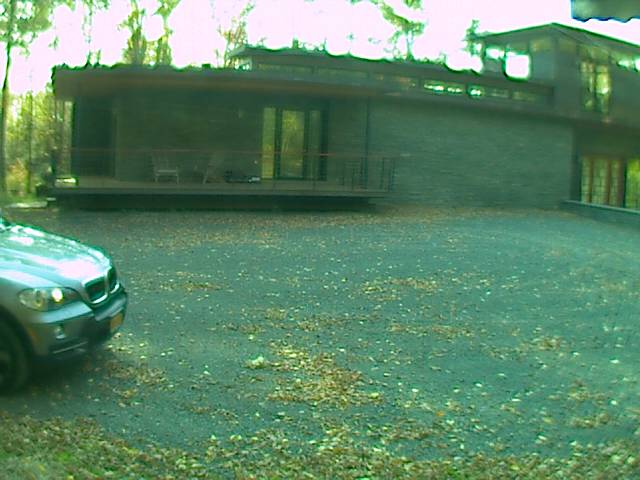The image captures a serene backyard scene of a brick, modern-style home. On the left side, the hood and front wheel of a silver car are partially visible. The well-maintained lawn is covered in small, fall-colored leaves that add a touch of seasonal charm. The house features rectangular architectural elements and large windows. A wrap-around porch with a sliding door offers a cozy outdoor space. Two brown Adirondack chairs are placed invitingly on the porch. Sunlight filters through the trees in the background, casting a warm, golden glow over the scene.